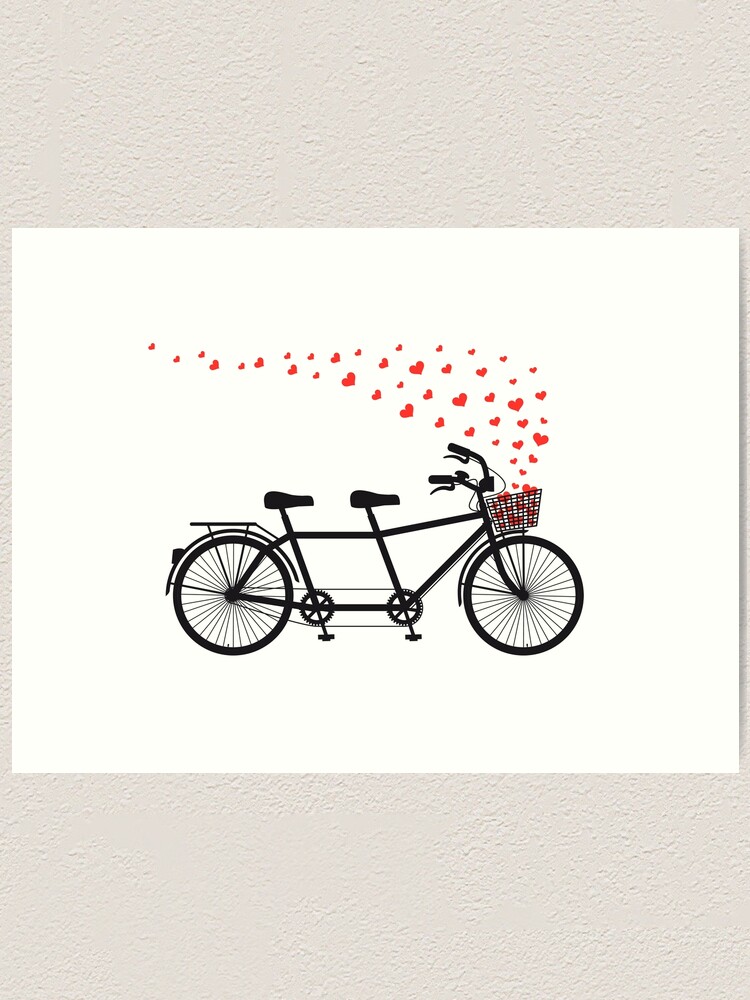The image depicts a black line drawing of a tandem bicycle, prominently situated at the center of a small, rectangular, white canvas, reminiscent of a piece of cardstock. The bicycle is depicted in a classic beach cruiser style, identifiable by its overly curved handlebars and low seats. A metal basket is affixed to the front of the bicycle, from which various sizes of valentine's red hearts cascade upwards and trail intricately towards the back, suggesting motion or wind. Enhancing its detailed realism, the bicycle features double brakes, individual pedals and gears, a guard on both the front and back tires, a light, and a small platform above the rear tire. The vivid red hearts are the sole splash of color against the monochrome drawing, creating a striking visual contrast. The image is devoid of any human figures or text, accentuating the whimsical charm of the floating hearts and the tandem bicycle.